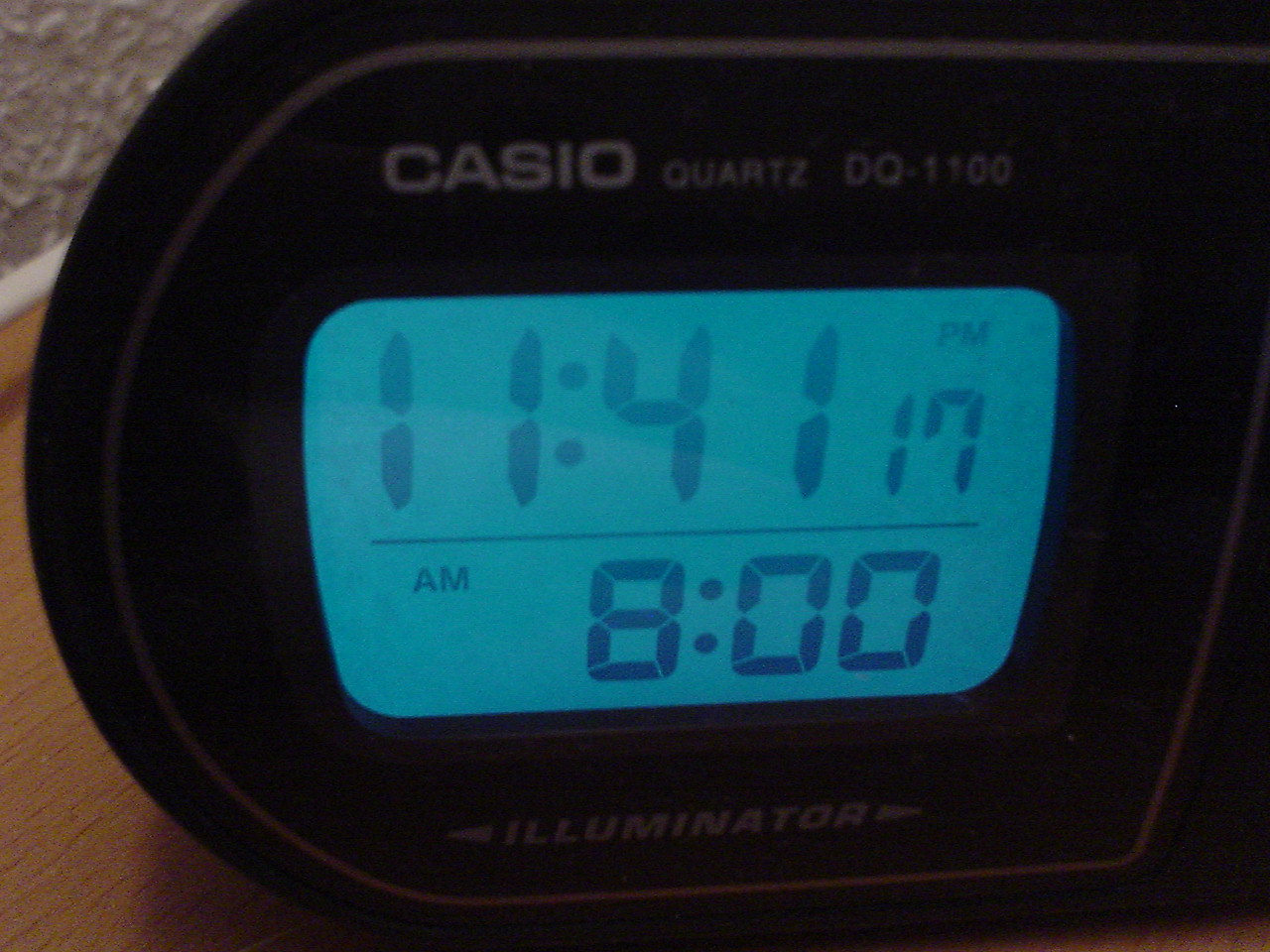A Casio Quartz DO-1100 bedside clock is prominently displayed in this photograph. The clock features a sleek design with a straight edge on the right and a gently curved contour on the left. The top of the clock is branded with "Casio Quartz DO-1100." Its blue square digital screen vividly displays the time as 11:41 PM and indicates an alarm set for 8 AM. The screen is bordered by the term "Illuminator," flanked by arrows pointing left and right. The clock is accented with a tasteful brown trim around its exterior and rests on a wood grain surface. The background consists of a textured stucco wall, adding an element of rustic charm to the scene.